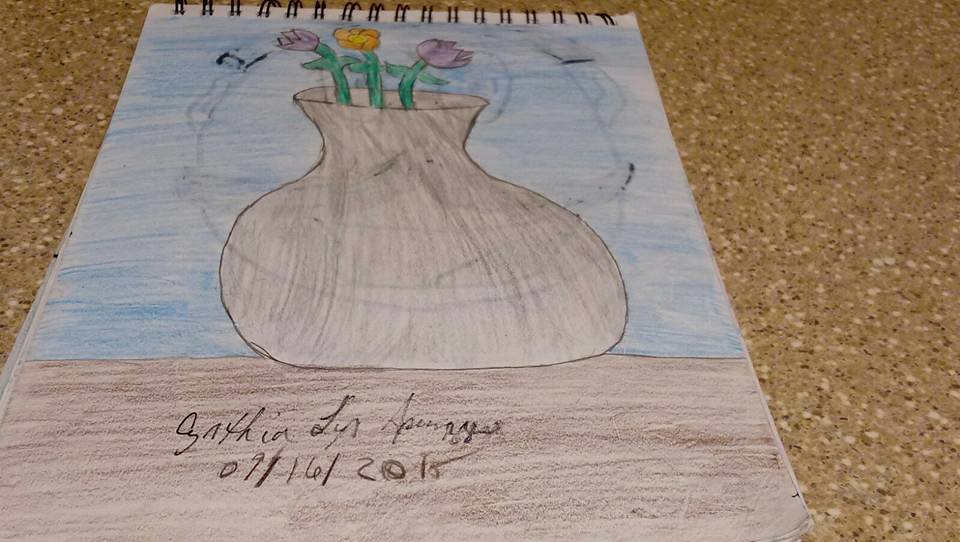In the photograph, a spiral-bound sketchbook, featuring black spirals at the top, rests on a speckled granite countertop. The open page reveals a striking artwork depicting a gray flower vase positioned on a brown surface. Emerging from the vase are three flowers: a purple tulip on the left, an orange flower with a yellow center in the middle, and another purple tulip on the right. The flowers have lush green stems and are set against a blue background, creating a vivid contrast. At the bottom of the sketchbook page, the artist's signature is inscribed along with what appears to be the date "09-16-2015".